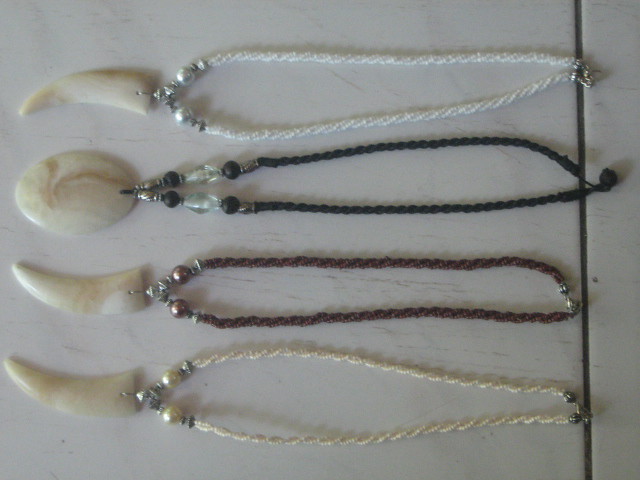This image depicts four horizontally arranged necklaces on a light tiled surface with thin, dark-colored marbling and a dark-colored grout line visible on the right side. Each necklace features a cord with beads and a distinctive carved pendant. The top necklace has a white cord with a tooth-shaped, possibly ivory dangle. The second necklace features a black cord with an oval-shaped, marble-like pendant. The third necklace consists of a brown cord with another tooth-shaped dangle, resembling a canine tooth. The bottom necklace displays a cream-colored cord and also has a tooth-shaped pendant. All the pendants are white and appear to be carved from similar material. The necklaces could be perceived as handcrafted, potentially mimicking traditional or ancient jewelry designs, and the photo suggests they might be listed for secondhand sale, possibly on a platform like Facebook Marketplace.